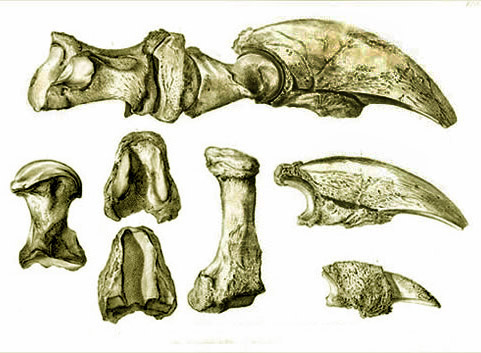The image is a detailed color illustration of several prehistoric bones, predominantly displayed in sepia tones against a white background, with light gray borders along the top and bottom edges. A large horizontal bone stretches from the top left to the top right corner, exhibiting a greenish-brownish-white color blend. This primary bone segment appears connected to a notable, large claw-like structure on the right, resembling the beak of a bird, likely indicating it’s part of an ancient dinosaur. Below the main bone are individually illustrated parts: a vertically oriented smaller bone to the left, two identical curved bones positioned centrally in the second row, and various other segmented bones including another claw and leg components arranged on the right side, providing a comprehensive anatomical breakdown. The illustration emphasizes the bones' intricate details and their connective features, suggesting it is a highly informative depiction of a prehistoric animal’s skeletal structure.